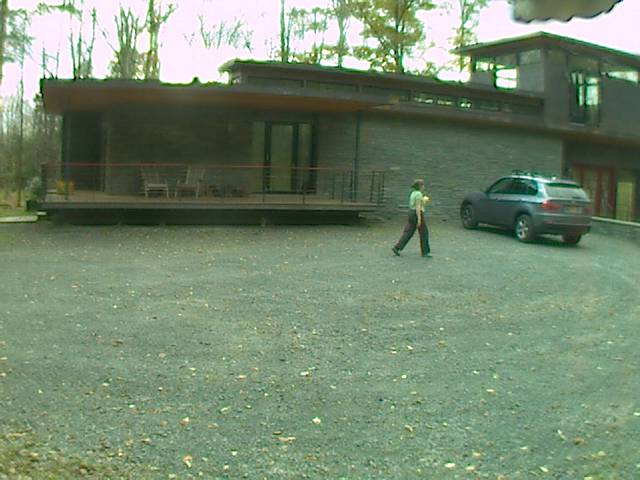This is a detailed photograph of a mid-century modern house featuring a distinctive architectural style with flat roofs and tall windows. The house is primarily ranch-style but includes a second story on the right side. A large awning covers a spacious porch area that spans one section of the house and is furnished with two Adirondack chairs. In front of the house, there is a wide, gray gravel driveway where a blue station wagon is parked.

A person is captured walking on the gravel driveway, appearing to be a Caucasian woman with her hair tied back in a bun. She is wearing a green short-sleeved shirt and long dark pants, and she holds a yellow object in her hand. The backdrop includes tall green trees indicating a daytime setting, with scattered leaves on the ground.